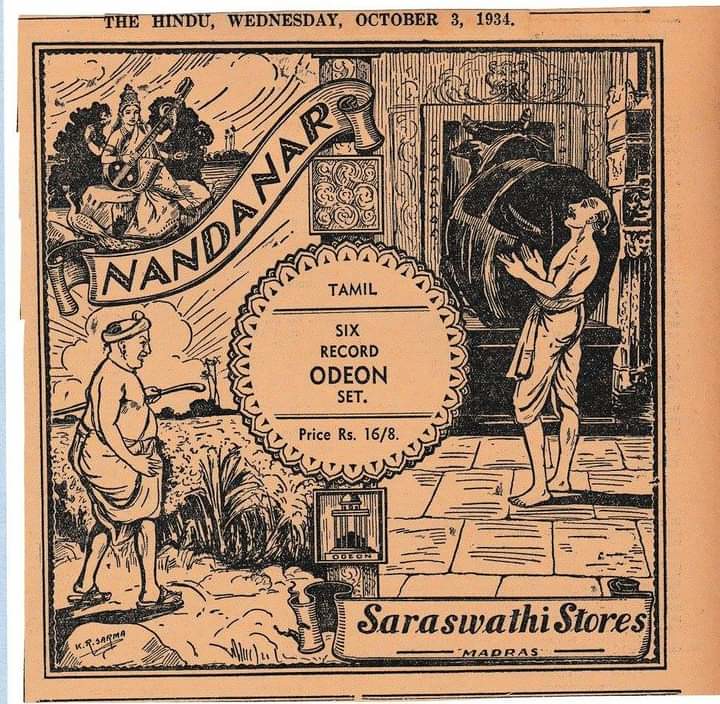This square, vintage color image, primarily in pale orange with black ink, appears to be a record album cover or an old booklet cover. The background evokes a nostalgic feel, with its classic design elements. At the top, it prominently states, "The Hindu, Wednesday, October 3rd, 1934," in white text. Towards the top left, written on a scroll-like design, is the word "Nandanar" (N-A-N-D-A-N-A-R). Centrally featured is a circular emblem with petal-like details surrounding it, containing the word "Tamil" (T-A-M-I-L). Below this, it denotes a "Six Record Odeon Set" (O-D-E-O-N) with a listed price of "R-S 16-8." In the bottom right, the text reads "Saraswathi Stores, Morris, Madras" (M-A-D-D-R-A-S). The image is crowded with intricate black-and-white sketches: in the top left, a person is depicted sitting on a rock playing a sitar; underneath, there's another figure in sandals tending to his crops outdoors. On the right side, a barefoot man stands on tiled flooring, adding to the rich cultural tapestry illustrated on this cover.